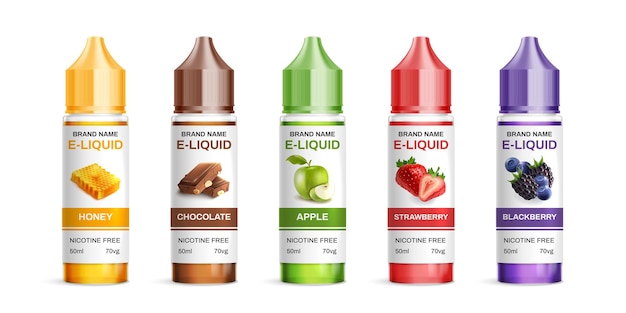This image depicts five cylindrical e-liquid bottles from a single brand, each arranged in a row from left to right. The bottles are uniform in shape, with cylindrical bodies and slightly curved tops that have a flat part. The bottles are different colors: yellow for honey, brown for chocolate, green for apple, red for strawberry, and purple for blackberry. Each bottle features a white label with "Brand Name" written in black at the top. Beneath this, the word "e-liquid" is displayed in the same color as the bottle. Each label also includes a corresponding image: a honeycomb for honey, a chocolate bar for chocolate, apples for apple, strawberries for strawberry, and blackberries for blackberry. Additional details indicate that the e-liquids are nicotine-free, each containing 50 milliliters, and have a 70 VG concentration, although the acronym VG is not defined in the image. The bottles' colors and glossy finish make them visually appealing.